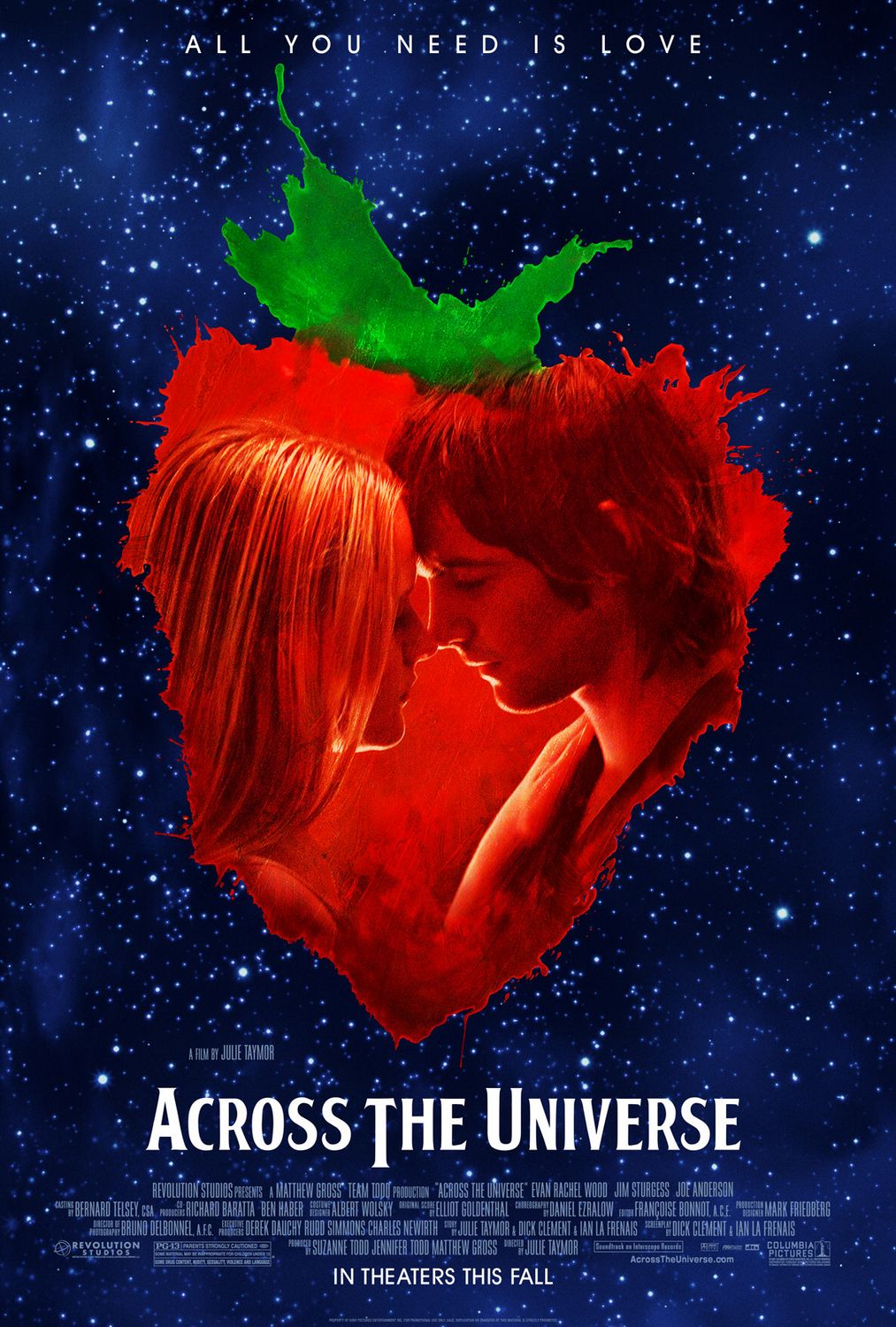This movie poster for "Across the Universe," directed by Julie Taymor, features a prominent, heart-shaped apple or strawberry outline in the center. Enclosed within this outline are the heads of a man and a woman, positioned intimately as if about to kiss, with the woman on the left and the man on the right. The background is a star-filled night sky adorned with hues of blue, black, white, and gray, contributing to a dreamy, cosmic ambiance. At the top of the poster, the text reads, "All you need is love." The bottom of the poster displays the movie title, "Across the Universe," along with the release information, stating it will be "in theaters this fall." The overall style and layout suggest this is an evocative and visually striking movie advertisement.